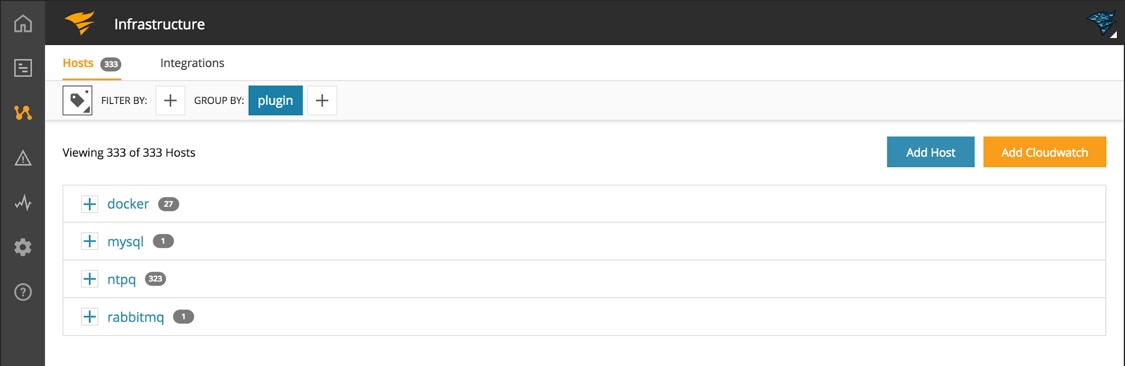In this screenshot, the word "Infrastructure" is prominently displayed at the top. An orange logo resembling a burning flame emanating from an arc is positioned next to it. The sidebar features several icons:

1. A house at the top.
2. A document below it.
3. A network node, resembling a share button, in the third position.
4. A triangle with an exclamation mark inside it in the fourth spot.
5. A line chart in the fifth position.
6. A gear icon next.
7. A question mark inside a circle at the bottom.

The main frame of the page is organized with two tabs at the top labeled "Hosts" and "Integrations." Below these tabs, there are buttons for filtering and grouping data, along with a prominent blue button labeled "Plug In." Black text below this button indicates, "Viewing 333 of 333 hosts." Two additional buttons, "Add Host" and "Add Cloud Watch," are located further down. This setup provides a clear and organized interface for managing infrastructure elements.